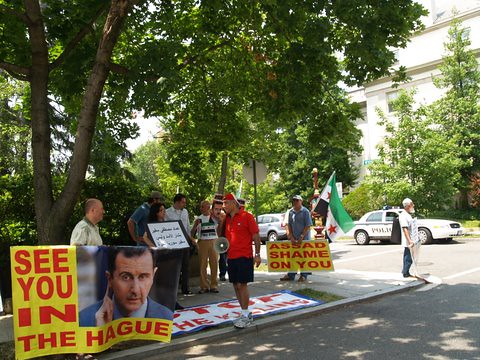In this daytime image, captured outdoors on a sunny day, a group of protestors is gathered on a busy street corner. Centered prominently in the scene are several individuals holding up various signs as part of a demonstration. The focal protest sign reads, “Assad, shame on you,” in bold red letters on a yellow background, while another banner states, “See you in the Hague,” suggesting this is an anti-Assad protest. Among the demonstrators, a man with a megaphone can be seen, alongside others holding placards and flags, including one with a green, white, and black design with red stars. The group includes both males and females, one notably a woman in a red t-shirt and black shorts holding a microphone. To the right, the scene extends into a road where police cars are parked near a white building. The leafy trees, casting their shadows on the pavement, frame the backdrop along with some distant cars and additional buildings, all under a clear sky that adds brightness to the protest setting.